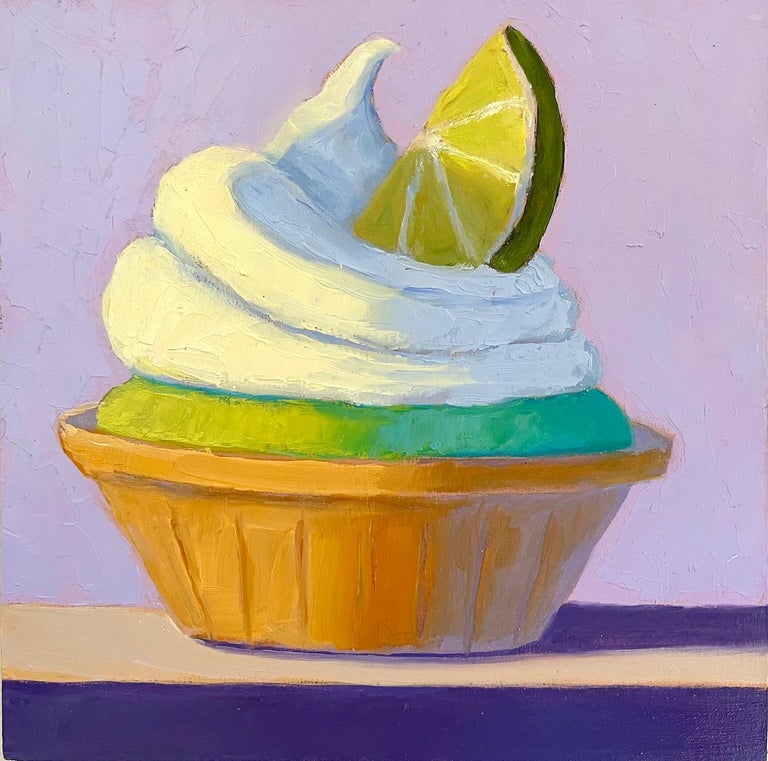This is a detailed painting of a green cupcake, housed in a light brown cup or wrapper. The green cake is topped with a thick, swirly puff of white whipped cream, intricately painted to reveal thick brush strokes indicative of oil layers. Nestled within the whipped cream is a lime wedge, adding a vibrant touch to the composition. The background features a light purple or lavender color, lending a soft contrast to the cupcake's vivid hues. The cupcake sits on a brown table, which bears purple shadows, enhancing the depth of the scene. The lime wedge is detailed with visible rind and subtle highlights, further contributing to the lifelike quality of this art piece.